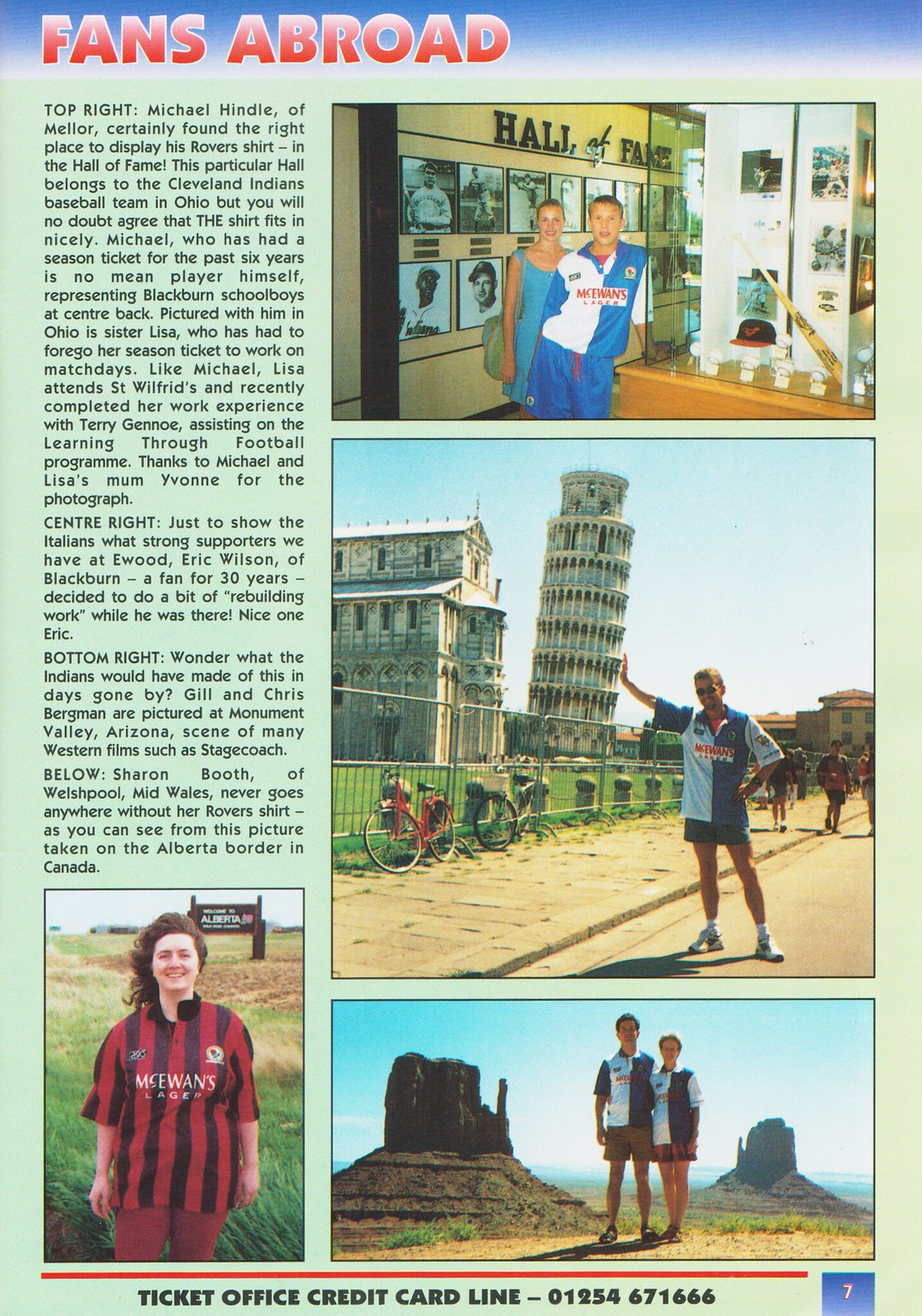The image depicts a vibrant poster titled "Fans Abroad" from a sports magazine, featuring passionately dedicated fans in various global locations showcasing their Rover shirts. The layout includes a light blue header with red font, and on the left-hand side, detailed descriptions of the highlighted fans. 

On the right-hand side, there are four distinct pictures. The top-right image shows Michael Hein of Mildred and his sister Lisa proudly displaying his Rover shirt at the Cleveland Indians Baseball Hall of Fame in Ohio, standing by a trophy case. Below this, a man poses cleverly at the Leaning Tower of Pisa, making it look like he's holding up the iconic structure with his hand. Further down, a couple donned in their ball jerseys stand against the expansive backdrop of a desert, possibly Utah.

On the left, a photo captures Sharon Booth of Willsport, West Wales, never seen without her Rover shirt, posing near the Alberta border in Canada. Another picture here features a woman in a field wearing a black and red jersey with the inscription "McEwans" in white font.

In the bottom right corner of the poster, a distinct blue box with an orange number 7 adds a touch of color contrast. This visually cohesive and richly detailed poster beautifully celebrates Rover fans' loyalty and adventurous spirit across the globe.